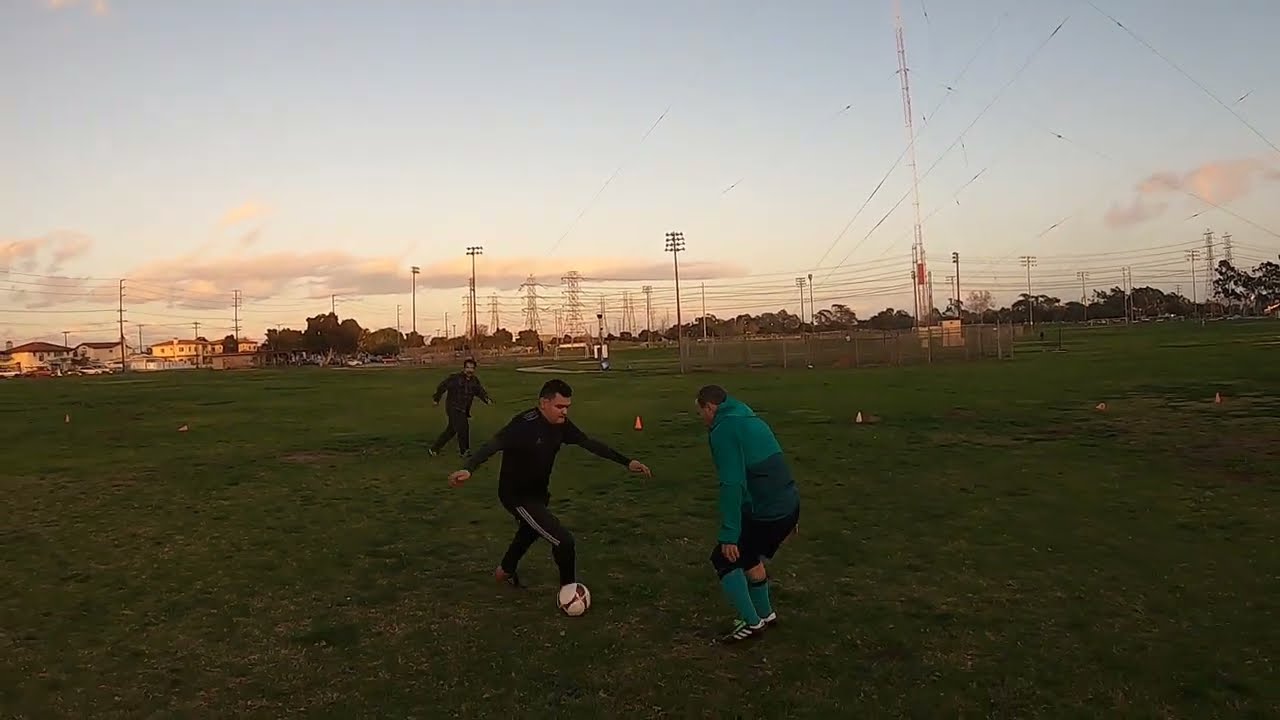In this image, two men are playing soccer in a large grass field as the sun begins to set, casting a slight orange hue across the minimally clouded sky. The man on the left wears a black jersey and black sweatpants with three white stripes along the side of his leg, while the man on the right is dressed in a green and blue sweatshirt, navy blue shorts, and green socks with blue at the top, complemented by black soccer shoes with three white stripes. The players are actively engaged, with the man in the green sweatshirt attempting to maneuver around the other. Nearby, orange cones are scattered on the field, indicating a practice session rather than an organized game, as there are no visible goals or drawn lines. Surrounding the field are numerous power lines and distant houses, though the immediate area remains an open space. The soccer ball they are using is white with red pentagons. Despite the approaching dusk, the field lights are off, and there is no text present in the image. The overall setting seems tranquil, capturing the essence of an informal yet spirited soccer practice.